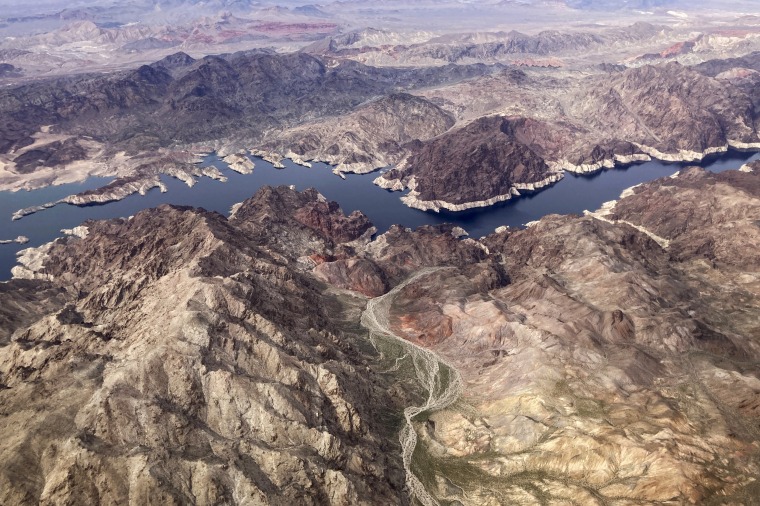This aerial photograph captures a strikingly rugged landscape, likely from the western U.S., with features reminiscent of regions like Colorado. The terrain is dominated by expansive, rocky hills with a somewhat cratered surface, displaying a varied palette of muted grays, browns, and blacks. Cutting through these jagged, uneven hills is a meandering waterway, whose still and deep blue waters provide a stark contrast to the surrounding earthy tones. This waterway, possibly a tranquil lake or river, acts as the only interruption in an otherwise endless expanse of stark, rocky terrain. No signs of human habitation, animals, or greenery appear in the scene, emphasizing the raw and untouched nature of this dramatic landscape.